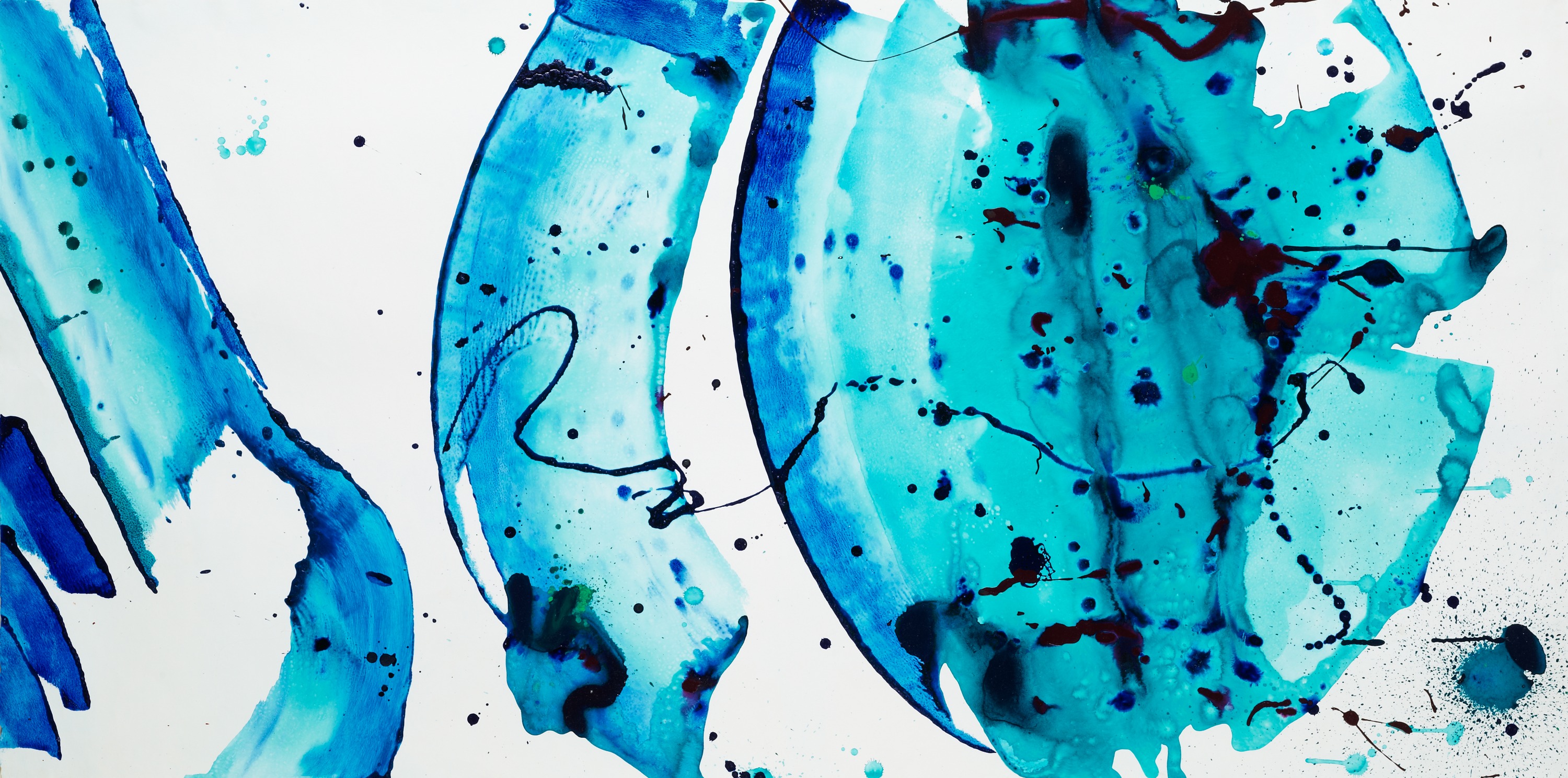In this abstract painting set against a white background, the primary focus is an egg-shaped blue splotch occupying the right section of the image from top to bottom. The main hues are various shades of blue, ranging from light turquoise to dark blue, with black ink blot-like splotches reminiscent of a Rorschach test pattern. To the left of the central blue oval, there's a rounded, cylindrical object with similar colors and splotches, curving slightly to the left. Further left, there is another elongated form that extends into a smaller, branching element; this too shares the blue tones and dark splotches but features fewer splotches overall. Near the lower left corner, there are three dark blue splotches standing out against the lighter background. Additionally, the lower right corner contains a small blue blotch and a black spot. Scattered throughout the image are smaller paint splatters, applied vigorously to create a dynamic appearance, reminiscent of Jackson Pollock's style. No text is present in the image.